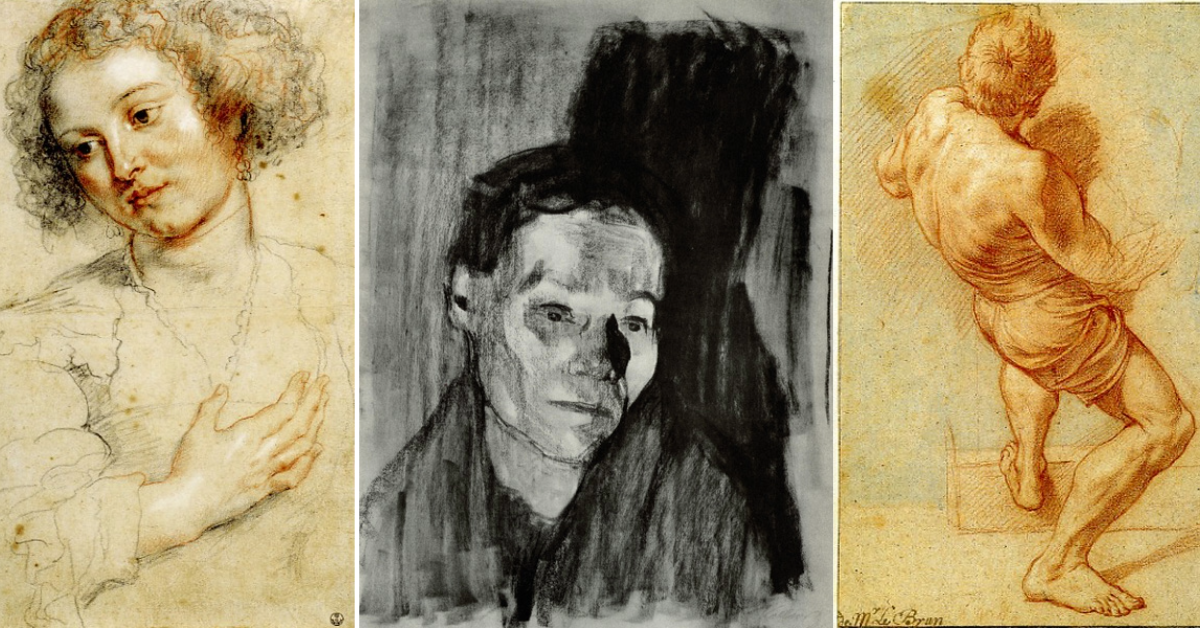This detailed drawing consists of three distinct, side-by-side images, separated by a white line, forming a cohesive collage that appears either sketched or painted. The left image features a woman with curly, hand-drawn hair that exhibits shades of reddish brown. She is depicted looking slightly downwards with her eyes open, her right arm across her chest. She wears a V-neck shirt adorned with multiple lines, suggesting a textured fabric. Her face, partially shaded, bears a contemplative or neutral expression.

The central image is a black and white sketch of a man with short hair and a saddened expression. His beady eyes, nose, and mouth are distinct yet minimally detailed, emphasizing his mood. He appears to be wearing a charcoal-colored coat or robe, adding to the somber atmosphere. His posture, slightly slumped, suggests introspection or melancholy.

The rightmost image portrays a muscular man with his back partially turned to the viewer, evoking a heroic or mythological figure akin to Hercules. He is shirtless, donning a skirt-like garment or fabric shorts, with bare muscular legs. His short hair complements his robust physique, and he appears to be holding something indiscernible in front of him. The artist's signature can be seen in elegant black cursive at the bottom right corner, adding a final touch of authenticity to the composite artwork.